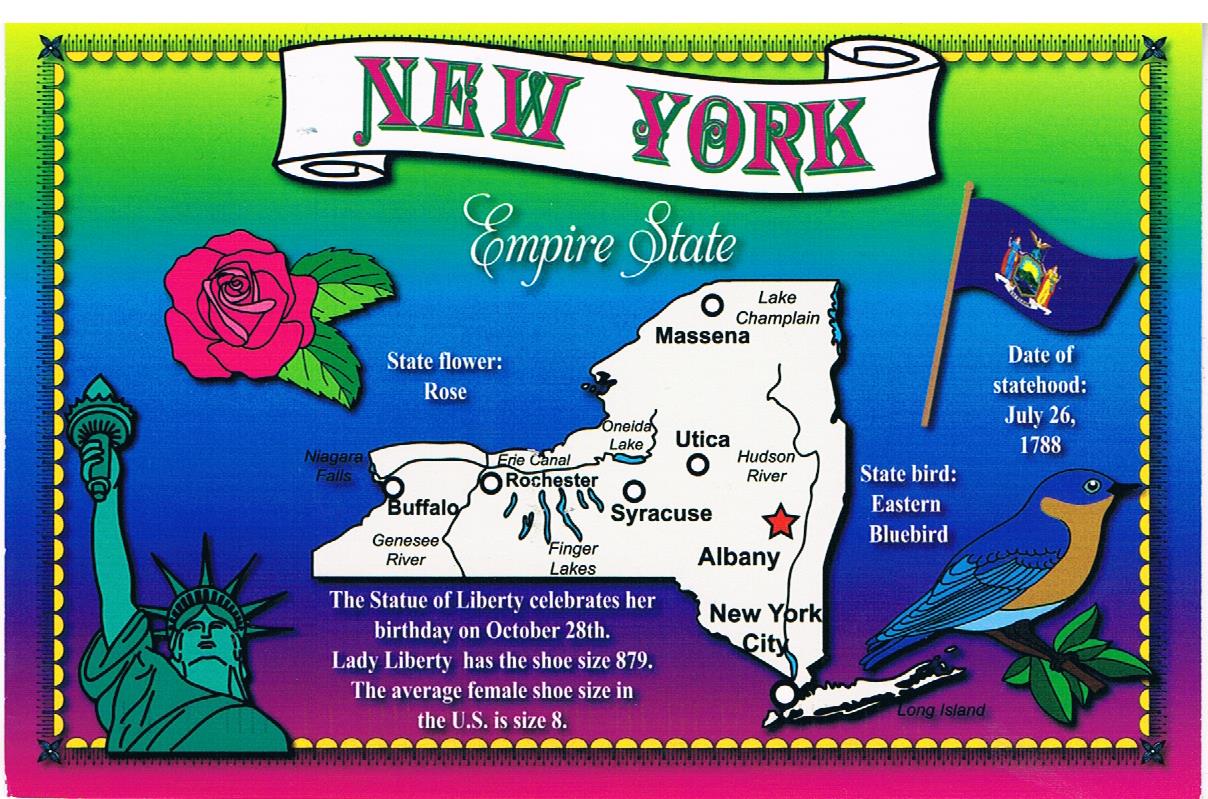This vibrant, postcard-like image showcases a whimsical, multi-colored tie-dye background with various elements celebrating New York State. Dominating the top is a decorative scroll banner in stylized green and pink text reading "New York, Empire State." Below it, a simplified map of New York State is centrally featured. The left bottom corner displays a cartoon depiction of the Statue of Liberty beside text noting her birthday on October 28th and her enormous shoe size of 879, contrasting the average U.S. female shoe size of 8. Adjacent to Lady Liberty, there's a striking red rose with two green leaves labeled "State Flower Rose." On the right side of the image, there's the New York state flag and its date of statehood, July 26, 1788, along with a detailed Eastern Bluebird perched on a branch with green leaves in the bottom right corner, labeled "State Bird Eastern Bluebird." The overall composition, rich in color and detail, offers a heavily collage-style homage to New York State with various shades of white, green, red, blue, and more interspersed throughout.